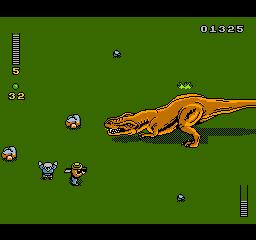This detailed color image depicts a screenshot with a predominantly green background, bordered by black sections at the top and bottom. In the top right corner, the number "01325" is displayed in a white font. On the left side of the top, a white ladder with black handrails is visible, bearing the number "5" beneath it. Directly below it is a green dot followed by the number "32."

In the bottom right corner, another white ladder with black rails appears, its purpose unclear. The central focus of the image is a tan-brown dinosaur, positioned with its head lowered and rear elevated. A drop shadow can be seen beneath the dinosaur, and its tail extends off the right edge of the screen.

Adjacent to the main figure, there are additional elements: two human-like figures, two balls in a yellow-peachy hue, and two blue balls. Additionally, an unidentified light green object is present. The composition of these various elements within the image remains ambiguous.